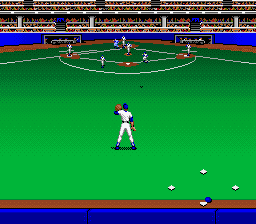This screenshot captures a nostalgic moment in a retro-style 2D baseball video game. The image is square-shaped and displays pixelated graphics reminiscent of older games. The scene is shown from a third-person perspective, focusing on a player in the middle of a vibrant green field. The player is dressed in a combination of a blue hat, blue undershirt, and a white uniform. They stand poised with their batting glove up, facing towards the empire. In the foreground, one can see the different bases with players positioned on them. Beyond the field, the stadium is partially visible, filled with spectators, though only the player with the mitt is rendered with detailed attention; the rest are more abstract. The overall composition evokes a sense of classic gaming charm.